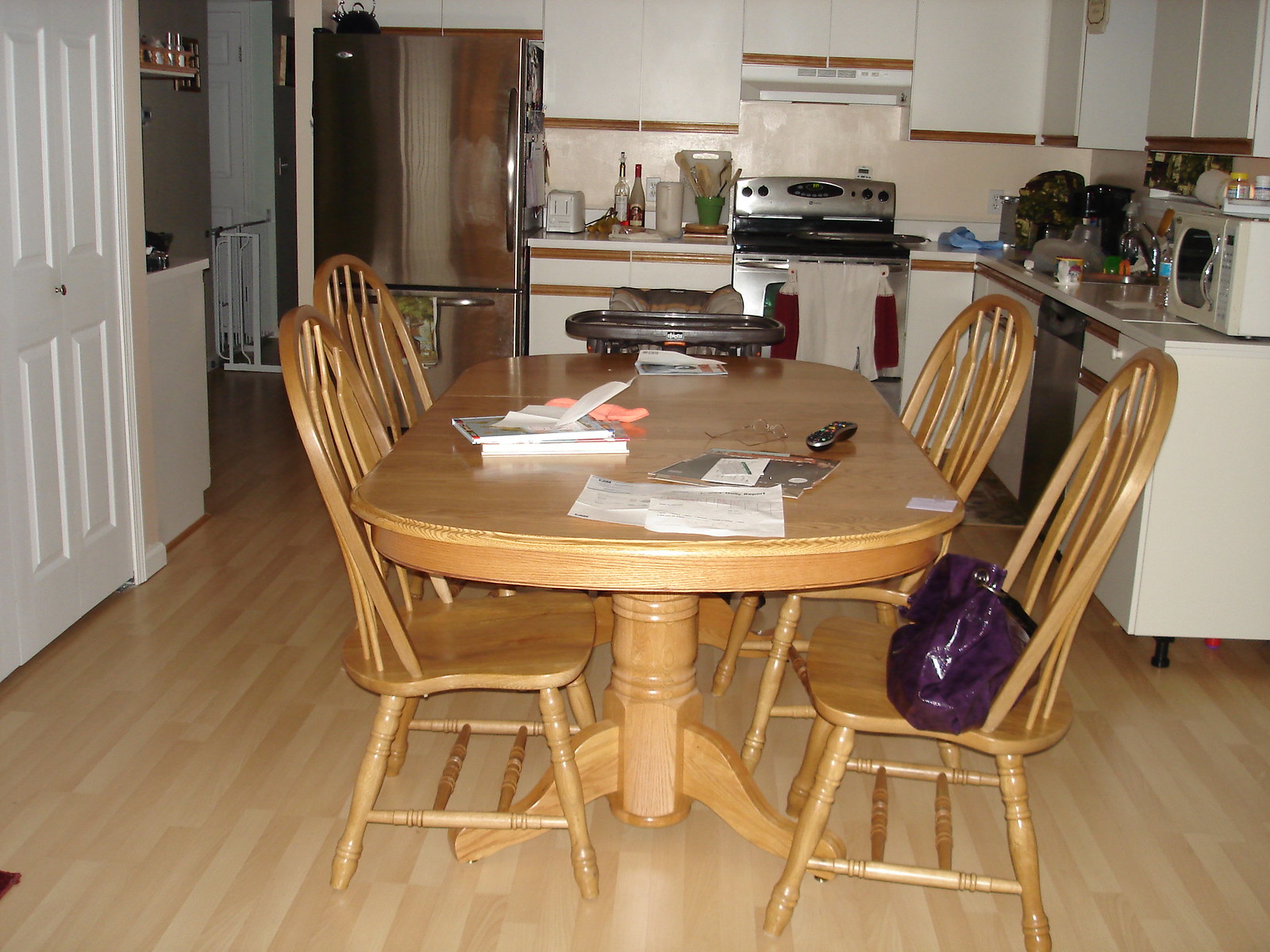This photograph captures a cozy kitchen and dining area, evidently taken with an older digital camera, lending it a nostalgic quality. Central to the scene is a light brown wooden table surrounded by four matching wooden chairs. The tabletop is cluttered with everyday items: a remote controller, a pair of glasses, several piles of papers, and a couple of books. At the table's end, a baby high chair is positioned, complete with a child's plate.

In the background, a sleek silver refrigerator stands next to the stove area. To the right, the kitchen sink and microwave are visible, flanked by countertops adorned with various utensils. A toaster, some bottles, a cutting board, and a cup filled with spoons are neatly arranged on the counters. On the left side of the image, a pantry door can be seen, and a baby gate is placed further back, marking the separation to another area. The detailed setup paints a lived-in and functional family space.